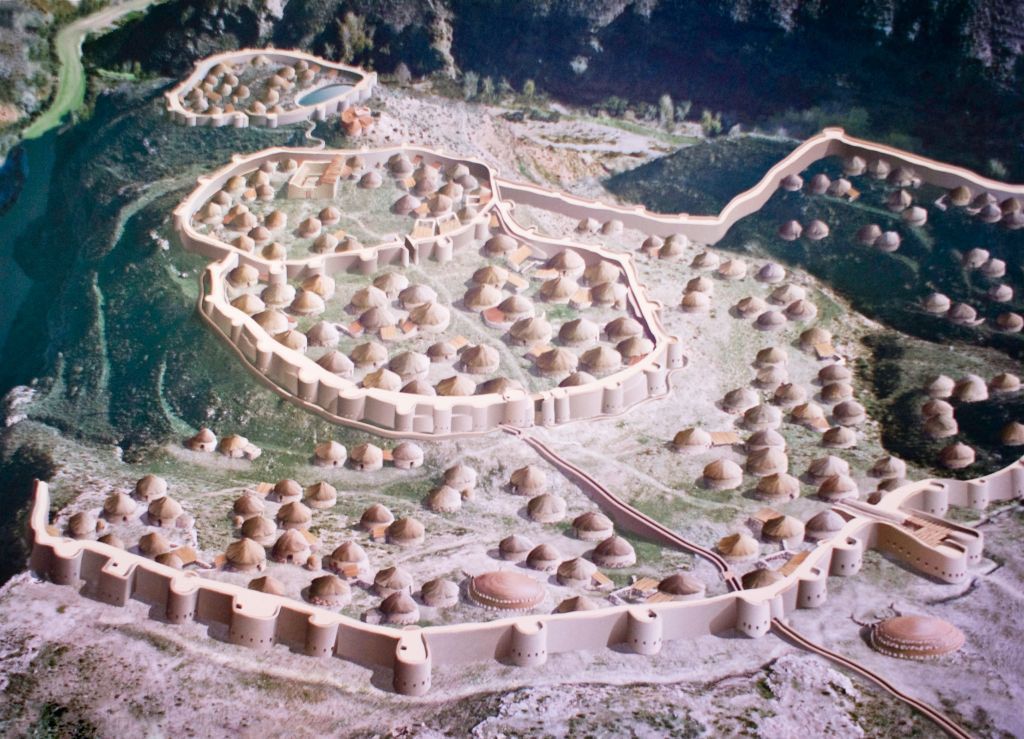A captivating aerial depiction of a fantastical settlement sprawls below, resembling a scene out of an elaborate dreamscape. The image provides a bird's-eye view, seemingly captured via a drone, showcasing a meticulously designed cityscape. Dominating the scene are numerous round-shaped huts or yurt-like structures, forming the core of this unique civilization. Encircling the entire settlement is a robust, thick tan-colored stone or brick wall, intricately weaving its way around the perimeter. This protective barrier also features multiple towers adorned with windows, providing vantage points across the wall.

The settlement's design suggests a complex hierarchy, as various zones within are also compartmentalized by similar stone walls, hinting at different sections or districts with specific purposes or status. Amidst the living quarters and walls, the landscape is punctuated by several patches of dark, verdant trees, adding a touch of natural beauty to the otherwise constructed environment. In the distance, majestic mountains loom, creating a dramatic backdrop that frames this enchanting world. The image captures not just a city, but a thriving, organized society nestled within a fascinating, otherworldly landscape.